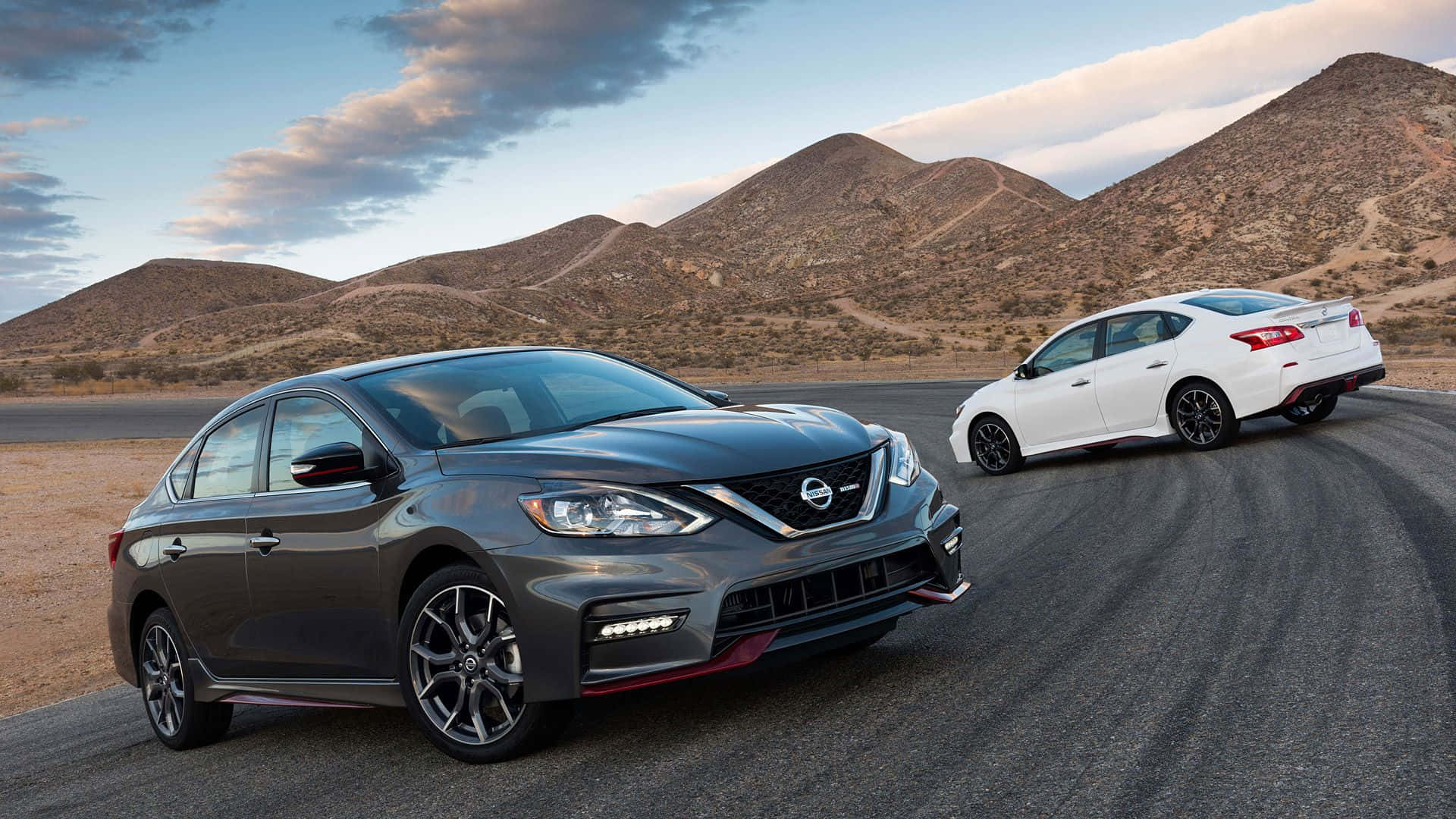This photograph is an advertising shot showcasing two Nissan sedans, positioned on a curving asphalt road that arches from the right foreground and sweeps to the left in the distance. The foreground features a solid gray Nissan with five-spoke rims, detailed with a red lip under the front, and a line of fog lights near the bottom. A solid white Nissan is parked further in the background, parallel but also diagonally positioned. Set in an arid, desert-like mountainous region with steep, non-craggy hills exhibiting dirt roads or trails, the landscape is dry and brown under a sunny, blue sky dotted with distant clouds. The cars, both four-door models, are placed almost perpendicular to the direction needed for driving, enhancing the dynamic feel of the scene. The blacktop road lacks any painted lines or markings, adding to the stark, rugged beauty of the setting.